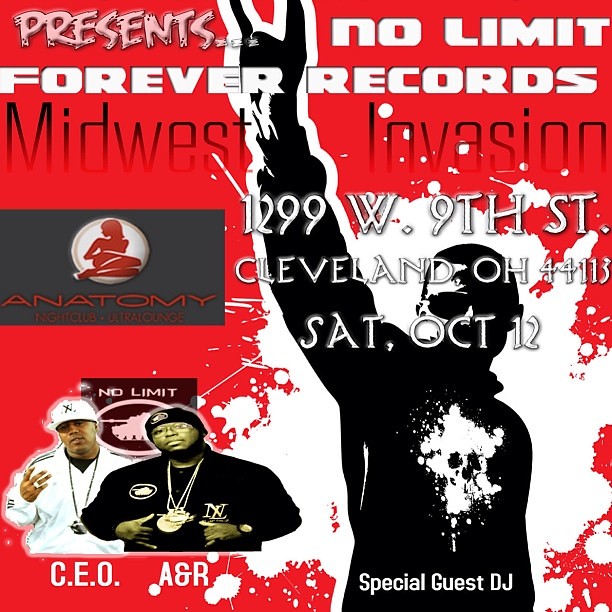The image is a promotional graphic for a nightclub event featuring DJs or rap artists, commonly seen on social media platforms. The background is predominantly red, accented with black and white. At the top, the white text reads "Presents No Limit Forever Records Midwest Invasion." Below this, the venue address "1299 West 9th Street, Cleveland, Ohio" is listed. The image features two frontal torso-up shots of male DJs or artists on the bottom left, labeled "CEO" and "A&R." CEO is clad in an all-white tracksuit with a black or white hat, while A&R is dressed in all black with a black beanie. To the bottom right, white text announces a "Special Guest DJ." Additionally, an impressionistic silhouette of a man, with pinky and index fingers extended and sporting sunglasses, is a notable visual element. Beside the artists, the logo for "Anatomy Nightclub Ultra Lounge" appears, anchoring the graphic's association with the event's location.